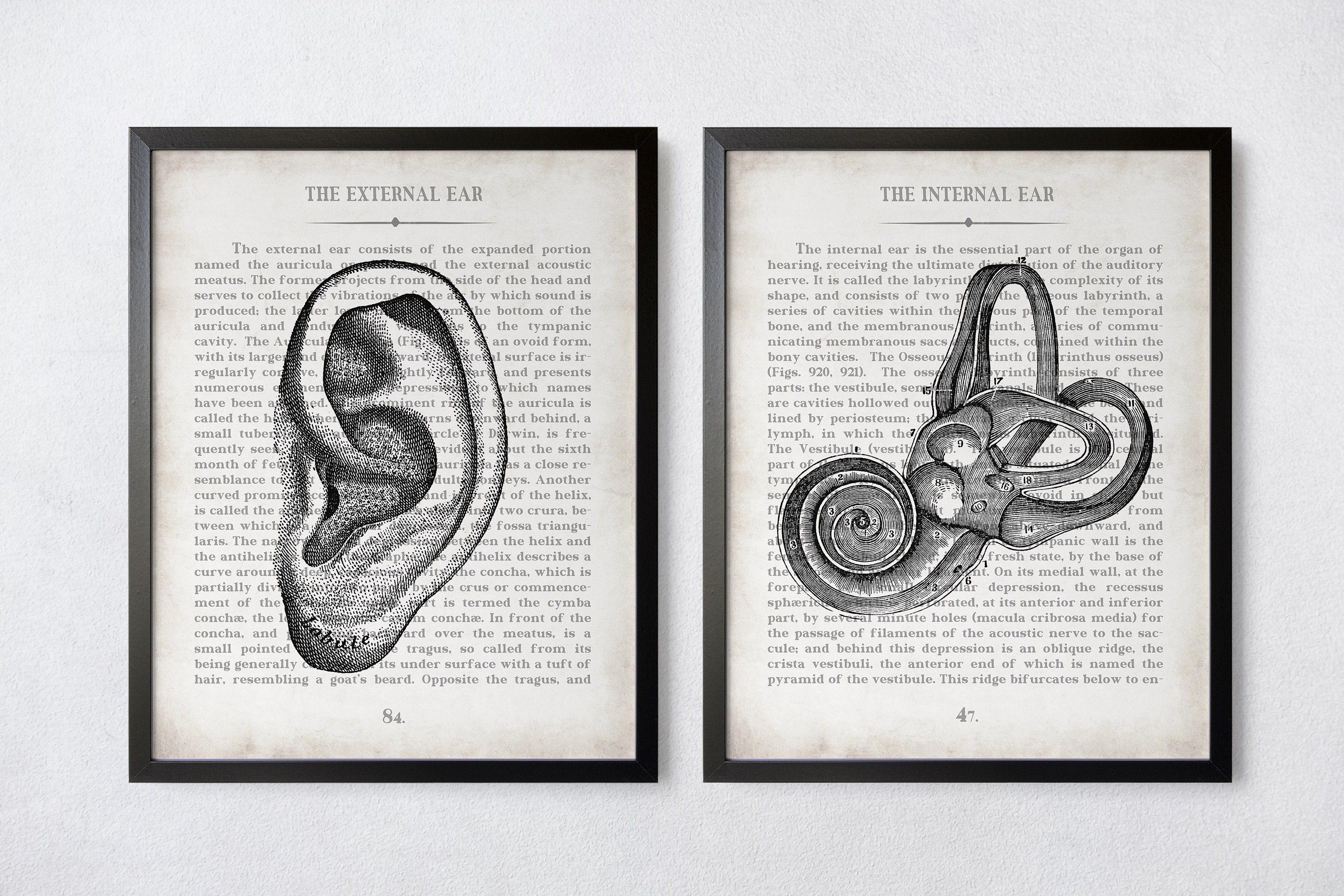The image showcases two framed pictures mounted on a white wall, each with a black border. The left frame is labeled "External Ear," featuring a large, pixelated drawing of an external ear made with tiny black and white dots. This picture is superimposed over a text-heavy background that is difficult to read but mentions detailed information about the structure and description of the external ear. The bottom of this frame displays the number 84. The right frame, labeled "Internal Ear," has a pixelated drawing of the internal ear, similarly detailed in pinpoint dots, showing its intricate parts, including a looped structure suggesting the ear canal. This image is set against another dense paragraph of text. The bottom of this frame is marked with the number 47. Both frames rest against a grayish-white background, suggesting they are hung on the wall for illustrative or educational purposes.